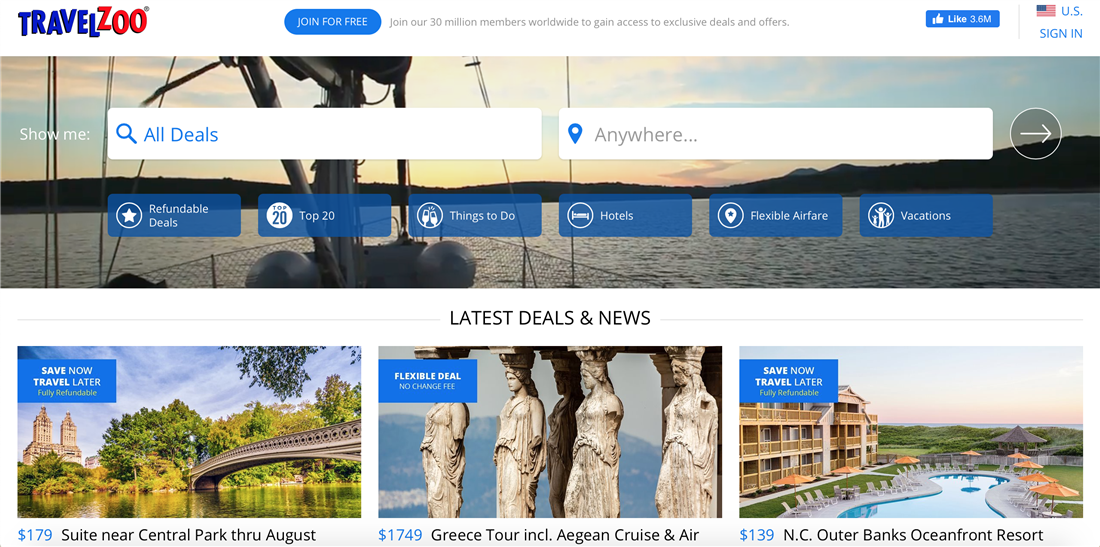This is a descriptive caption for an image of the Travelzoo website:

---

The Travelzoo homepage invites users to join its 30 million members worldwide for exclusive deals and offers, resembling a Facebook layout with a prominent "Like" button and 3.6 million likes. A "Sign In" option is displayed alongside a United States flag. At the top, a search bar allows users to explore deals or destinations by typing preferred locations. Various options are available under the search bar, including "Refundable Deals," "Top 20," "Things To Do," "Hotels," "Flexible Airfare," and "Vacations." 

Further down, "The Latest Deals and News" section promotes offers like a $179 suite near Central Park available through August, a $1,749 Greece tour with an included Asian cruise, and a fully refundable $139 stay at NC Outer Banks Oceanfront Resort, showcasing a pool adjacent to the ocean. A background image depicts female statues, many with broken arms, serving as columns for an ancient structure.